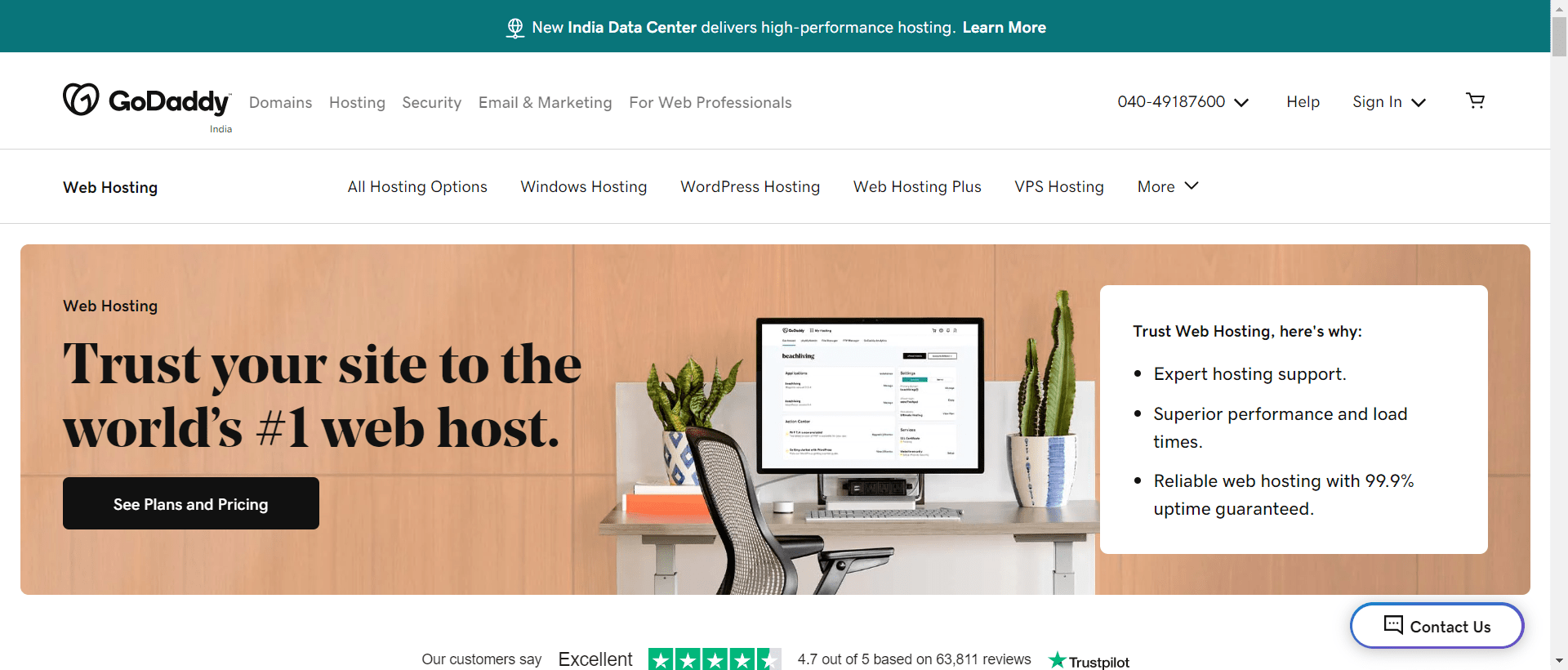The image is reminiscent of a horizontal splash page from GoDaddy aimed at marketing. At the top, a teal-colored horizontal bar reads, "New India Data Center delivers high performance hosting, learn more." Below this, from left to right, it lists various services: "GoDaddy domains, hosting, security, email and marketing for web professionals." To the right, a phone number "040-491-67600" is displayed with an arrow pointing downwards, indicating a dropdown menu. Adjacent to it are the options "Help" and "Sign in," each with downward arrows symbolizing dropdown menus. A shopping cart icon is positioned at the far right.

Beneath these elements, a horizontal menu offers additional services: "Web hosting, all hosting options, Windows hosting, WordPress hosting, web hosting plus, VPS hosting," with the word "More" accompanied by a downward arrow indicating a dropdown menu.

The main section features a box with a light brown paneled background, reminiscent of an office setting. On the left, it reads "Web Hosting. Trust your site to the world's number one web host," with a black rectangle below that says "See Plans and Pricing" in white text.

The central part of the image includes a small office cubicle setup. Two plants in blue and white planters are situated within the cubicle; the plant on the left is shorter and the one on the right is taller with large, flat, light and dark green leaves. Another plant resembling a cactus is also present. The office setup includes an ergonomic chair with a mesh back, a light gray metal desk, a keyboard, a monitor, and a mouse. The monitor is turned on, but the content on it is indistinguishable.

To the lower right, there is a blue-ringed oval button that says "Contact Us" in black. At the bottom center of the image, customer feedback is highlighted: "Our customers say Excellent," accompanied by green stars and a rating of "4.7 out of 5 based on 63,811 reviews." The section is concluded with a green star and the Trustpilot logo. No additional text is present.